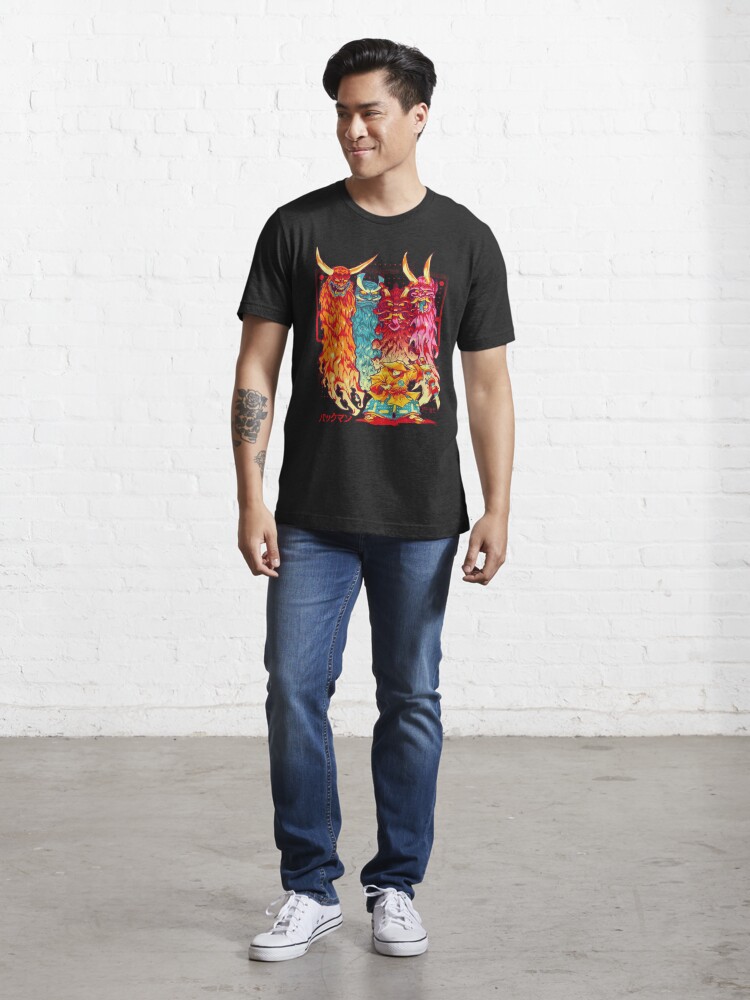This is a detailed portrait photograph of an Asian man, approximately 30 years old, standing at the center of the frame against a white-painted brick wall with a gray concrete floor. The background consists of about 70% white brick wall and 30% concrete floor. The man is wearing a black cotton short-sleeve t-shirt adorned with four colorful dragon-like creatures—one orange, one blue, one maroon, and one pink—all featuring cream-colored horns. His t-shirt also has a large flower design on the front. He is paired with blue jeans and white Converse sneakers. The man has short black hair, shaved on the sides and styled in a modern flip over the top, and he is smiling while looking to his right. Notably, he has a tattoo on his right forearm. The minimalist background and his poised stance give the impression that he might be modeling for a magazine or a catalog.